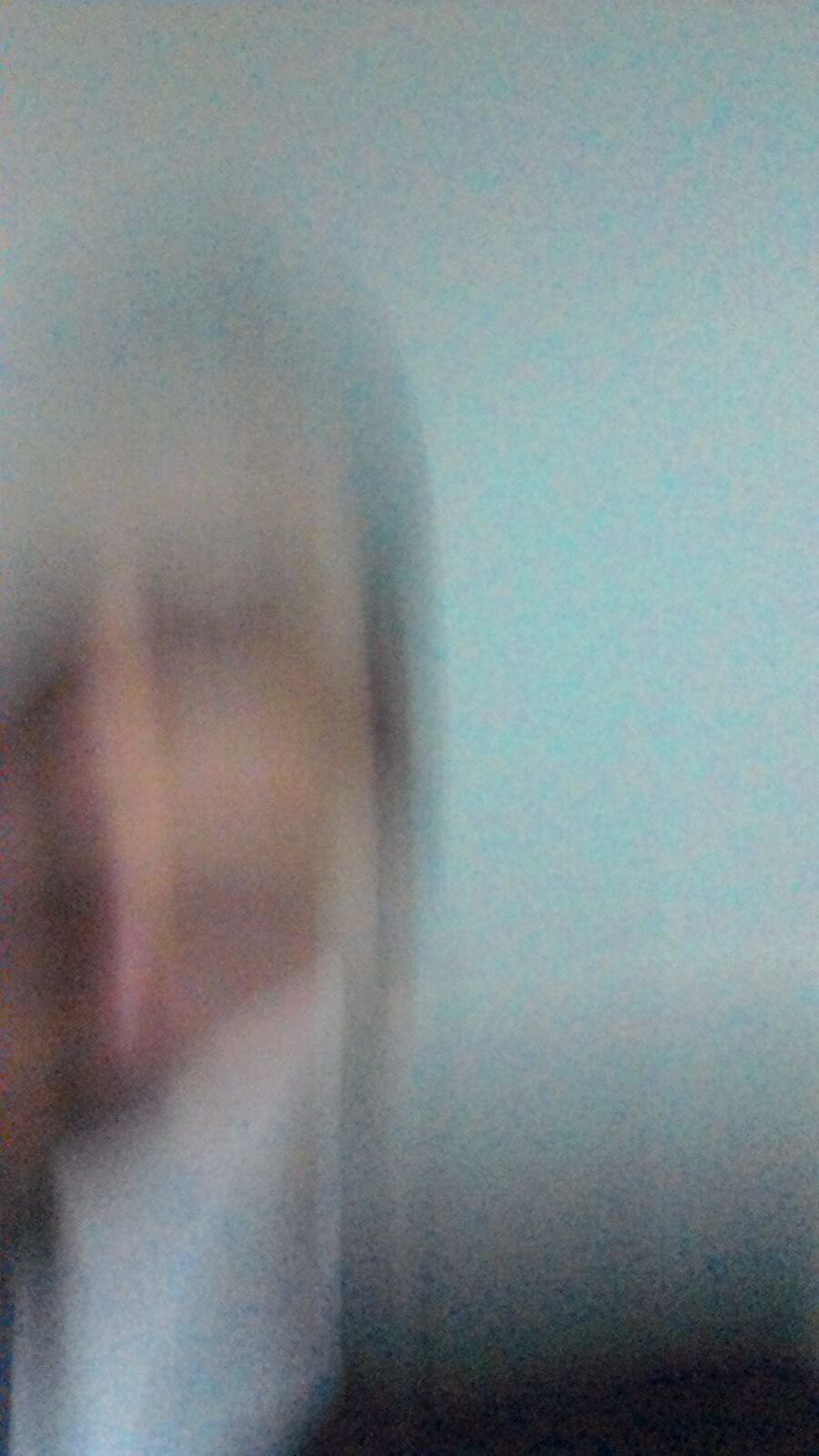The image portrays an extremely blurred and abstract depiction of what appears to be a person's face. The left side of the image suggests the presence of facial features, with a slightly discernible nose and hints of eyes partly visible through the distortion. The face seems to be framed by dark brown or black hair and possibly obscured by a white mask covering the mouth and part of the nose, adding an element of intrigue or anonymity. The right side transitions into a gradient of colors, starting from a mix of grayish and greenish hues and fading into a deep black towards the bottom right corner. This side provides a stark contrast to the suggestive figure on the left, contributing to an artistic, almost ethereal quality. The overall composition leaves much to the imagination, inviting viewers to ponder the identity and intent behind the blurred visage.